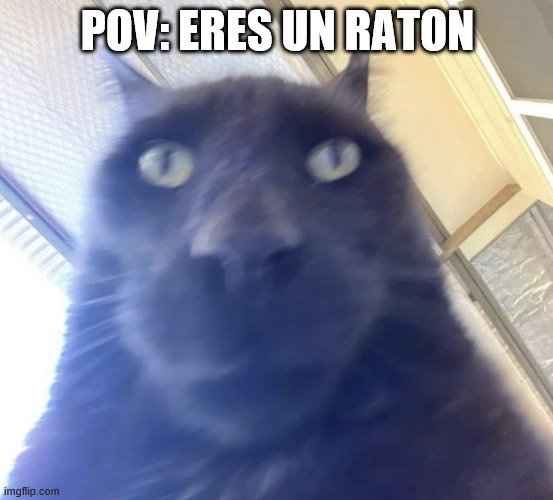The image features a close-up view of a black cat's face, taken from a low angle that distorts its appearance, giving the cat's face an exaggeratedly large effect. The cat's eyes are striking, with a clear note of green and black pupils. The photo has a slight blurriness which adds to the surreal, almost larger-than-life quality of the cat's face. The setting appears indoors, as suggested by visible elements in the background, including a tan-colored ceiling, a white wall, a shelf, and the top part of a window. On the top middle of the image, there is text in white that reads, "POV: Eres Un Ratón," hinting at a Spanish phrase. In the bottom left, the watermark "igmflip.com" is displayed in black. The overall color palette includes white, black, light green, off-tan, cream, and hints of silver, contributing to the indoor, somewhat casual atmosphere of the photo. The cat's ears are pointed up and it is looking directly into the camera.